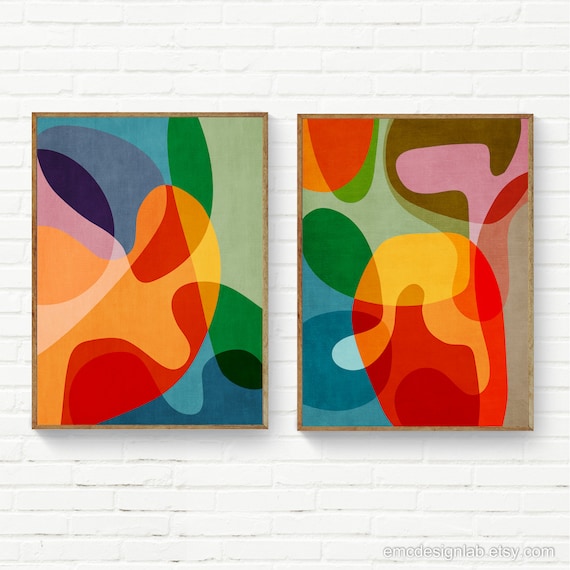This image features two framed abstract art prints mounted on a clean, white brick wall. Both pieces are bordered by narrow wooden frames and display swirling, layered splotches of vibrant colors. The left painting showcases an intricate mix of orange, pink, red, blue, green, and dark blue splotches, blending fluidly into one another to create new shades. Similarly, the right painting features a stunning mélange of red, blue, green, orange, brown, pink, and light blue hues, maintaining a cohesive yet slightly varied visual from its counterpart. The color blobs in both artworks meld in a way that mimics the smooth, rounded shapes you might find in a lava lamp, creating an effect of continuous motion and depth. Positioned high on the wall, the pieces are of equal size and shape, enhancing their unified presentation. At the bottom of the image, a website link—emedesignlab.etsy.com—suggests these prints are available for purchase, further indicating their potential as listings on Etsy.